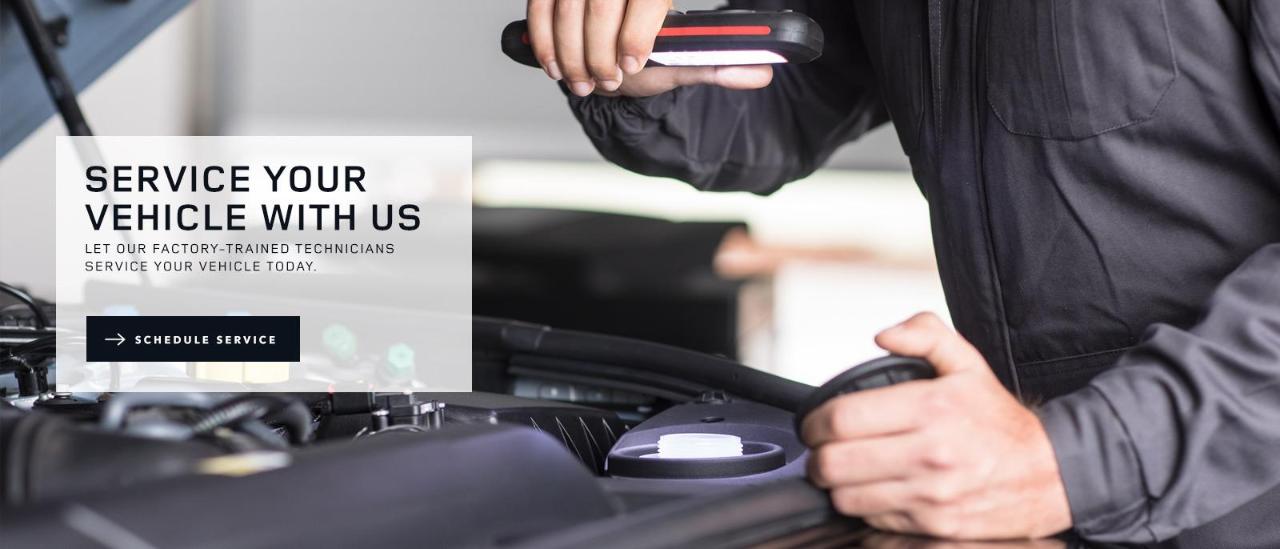The image captures a busy service shop environment. At the forefront, the chest and hands of a skilled service technician are visible. The technician, clad in a dark gray jumper coat, is holding a specialized instrument in his right hand and a removed vehicle part in his left hand. To the right, the hood of a vehicle is propped open with a visible black cladding. An extendable strut supports the hood, highlighting the intricate work being done. In the background, a slightly blurred message box stands out with the text, "Service your vehicle with us" in black lettering against an off-white backdrop. Below it, another line reads, "Let our factory-trained technicians service your vehicle today." At the bottom, a long black rectangle contains the words "Schedule service" in white lettering with an arrow, suggesting an action to be taken. The image focuses on the technician, emphasizing the precision and care put into vehicle maintenance.